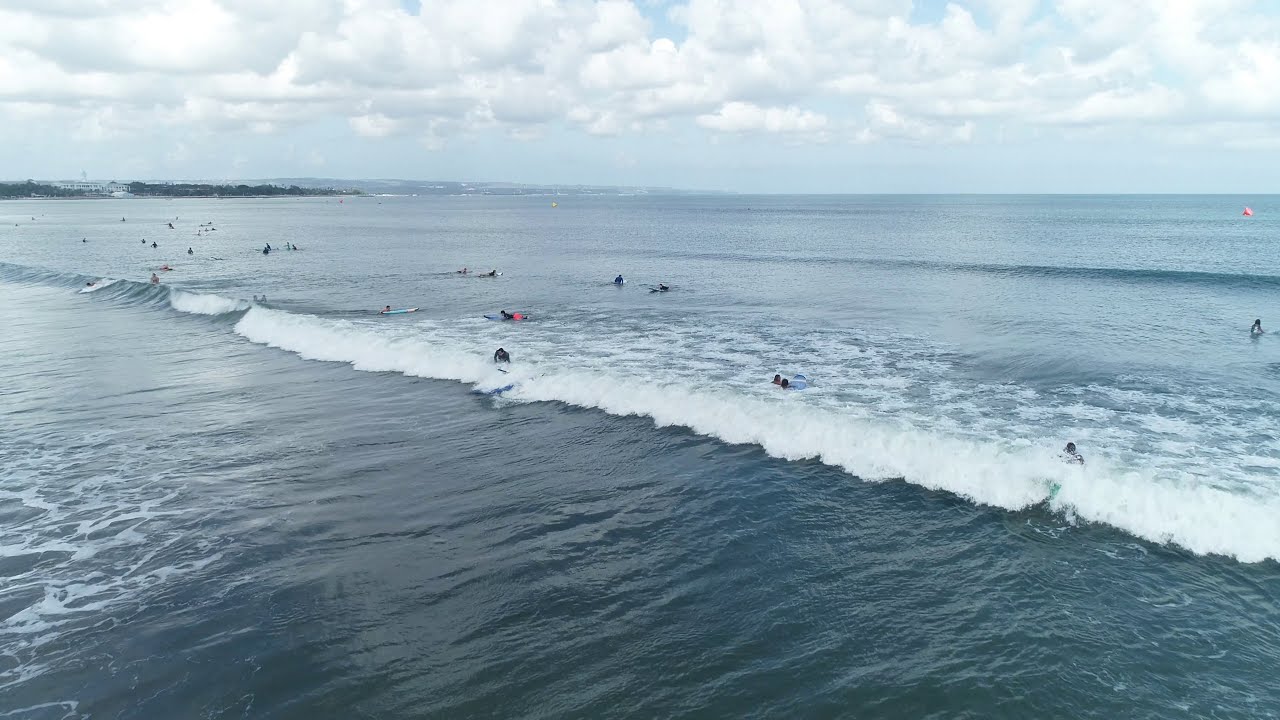This image captures a stunning ocean scene dominated by deep blue, expansive water. Approximately two-thirds of the image is occupied by this vast body of water. The horizon slices across the top third of the frame, leading into a light blue sky dotted with puffy, cotton ball-like clouds. In the midsection of the image, a prominent wave is breaking diagonally from the bottom right to the center left, forming white foam as it crashes. Along this wave, several people can be seen; some are swimming while others are riding surfboards or bodyboards. Further into the distance, more surfers are visible, sitting on their boards in calmer water. In the upper left corner, there is a hint of coastline with greenery and a few white buildings, adding depth to the scene. The tranquil backdrop of the sky, coupled with the vivid blue of the ocean and the dynamic movement of the waves, creates a captivating and lively seaside panorama.